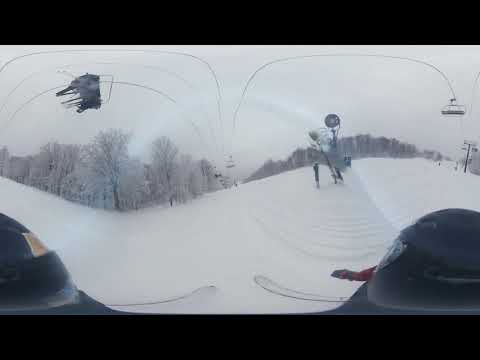This image, taken from the perspective of someone sitting on a ski lift, features a snowy hillside surrounded by trees blanketed in white. The picture is framed by black borders on the top and bottom, giving it an enclosed and focused look. The scene is slightly distorted, possibly due to a fisheye or panoramic lens, which adds to the perception of movement and depth.

In the foreground, the knees of the person capturing the image are visible, clad in protective gear, and their white skis jut out on either side. The foreground also includes two roundish black objects in the left and right corners, which appear to be the ends of the ski lift apparatus.

The middle of the image shows a twisted and somewhat surreal perspective of the ski slopes. There is a clearly defined path flanked by trees on both sides, leading towards the background. Tall light poles can be seen on the right side, adding an industrial touch to the otherwise natural setting. Above the trees on the left, a sideways image of a ski lift is evident, with its wires stretching up and over the scene. On the right, a single ski chair is suspended in the air, contributing to the overall sense of motion within the image.

In the center-right of the frame, a piece of dark gray machinery, possibly a snow-making machine, stands out, hinting that this location might rely on artificial snow. The day appears overcast, casting a gray hue over the entire landscape. This image encapsulates the serene yet busy atmosphere of a bustling ski resort, viewed through a unique, slightly distorted lens that captures the essence of the winter activity.